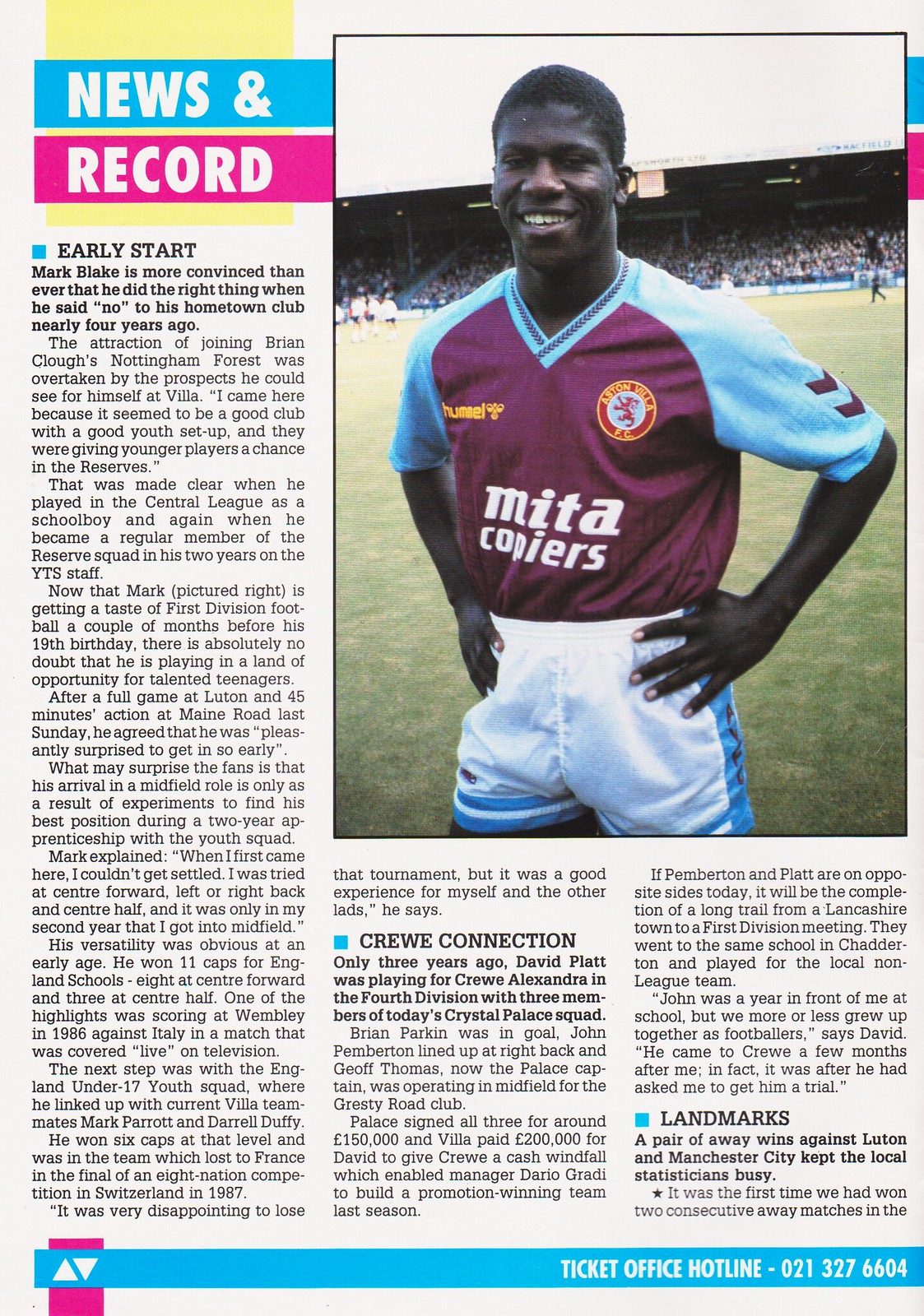The image depicts a detailed page from a soccer program, showcasing both a news article and a photo of an athlete. Dominating the upper right corner is a photograph of a smiling athlete, likely of African descent, standing confidently on a green soccer field in front of a stadium. He has dark skin, clean-shaven, and dark black hair. His uniform features light blue raglan sleeves and a maroon chest area emblazoned with "Mita Copiers" in white lettering. He wears white shorts with a matching blue stripe and poses with arms akimbo, exuding confidence.

The article itself is divided into three columns beneath the headline "News and Record," with "News &" in white lettering over a blue background and "Record" over a dark pink background, all on a pale yellow backdrop. Subtitled "Early Start," it discusses Mark Blake's decision to decline his hometown club offer nearly four years ago and expresses his growing conviction that he made the right choice. Interspersed within the main text are sections titled "Crew Connection" and "Landmarks," which mention David Platt’s past with Crew Alexandria and significant away wins against Luton and Manchester City respectively.

At the bottom of the page, a light blue horizontal bar contains the contact information for the Ticket Office Hotline, marked in white text at 021-327-6604. This blue bar is superimposed over a pink rectangular strip and features directional triangles on the left, adding visual elements to the layout.